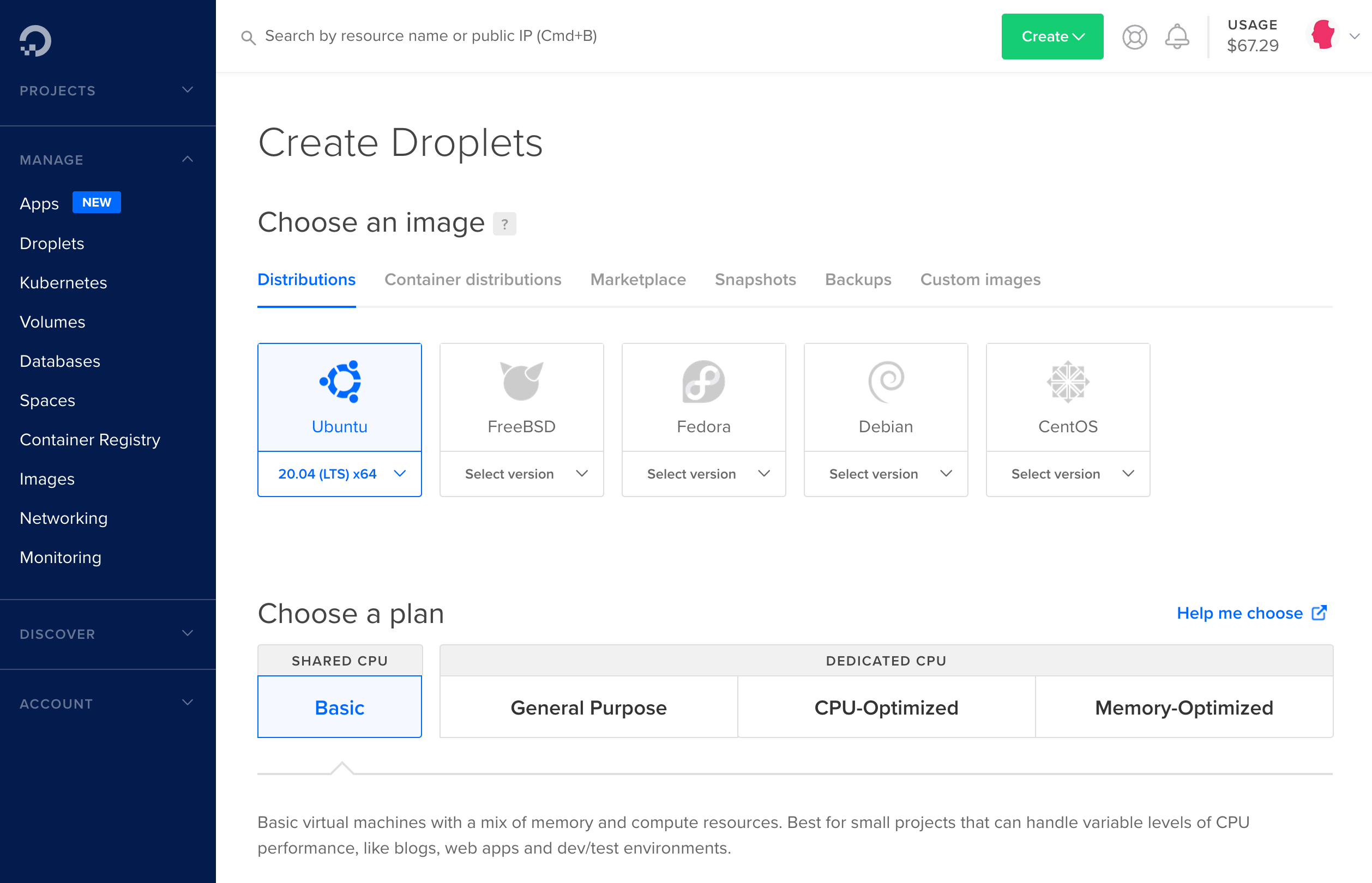In this detailed screenshot of a web management interface, the left side of the page features a dark blue menu with a selection of options including Projects, Manage, Apps, Droplets, Kubernetes, Volumes, Database, Container Registry, Images, Networking, Monitoring, Discover, and Account. Under the "Manage" section, there is a highlighted "Apps" option with a prominent blue "New" button.

On the top left, an "O" icon in grey is visible, while the right side of the page, set against a white background, displays a search bar with the placeholder text "Search by resource name or public IP CMT + B." To the right of this search bar, there’s a green "Create" button next to a usage information display that reads "USD 7.29."

Below the usage info and the create button area, the section titled "Create Droplet" is visible. Users are prompted to "Choose an image," with several tabs available for selection, such as Distribution, Container Distribution, Marketplace, Snapshots, Backups, and Custom Images. In this case, the "Distribution" tab is highlighted in blue. Within it, the Ubuntu distribution is also highlighted in blue, followed by other available distributions like FreeBSD, Fedora, Debian, and CentOS, each accompanied by a "Select Version" drop-down menu.

Further down, the page invites users to "Choose your plan," with various plans displayed. The "Shared CPU Basic" plan is highlighted in blue, while additional options listed include Dedicated CPU, General Purpose, CPU-Optimized, and Memory-Optimized plans. An option to get assistance, labeled "Help me choose," is written in blue on the top right of this section.

At the bottom of the screen, a detailed explanation describes the "Basic" plan under "Shared CPU," noting that basic virtual machines with a mix of memory and compute resources are best suited for small projects requiring variable CPU performance levels, such as web apps, development, and testing environments. The explanation directly references the "Basic" option within the Shared CPU plans.